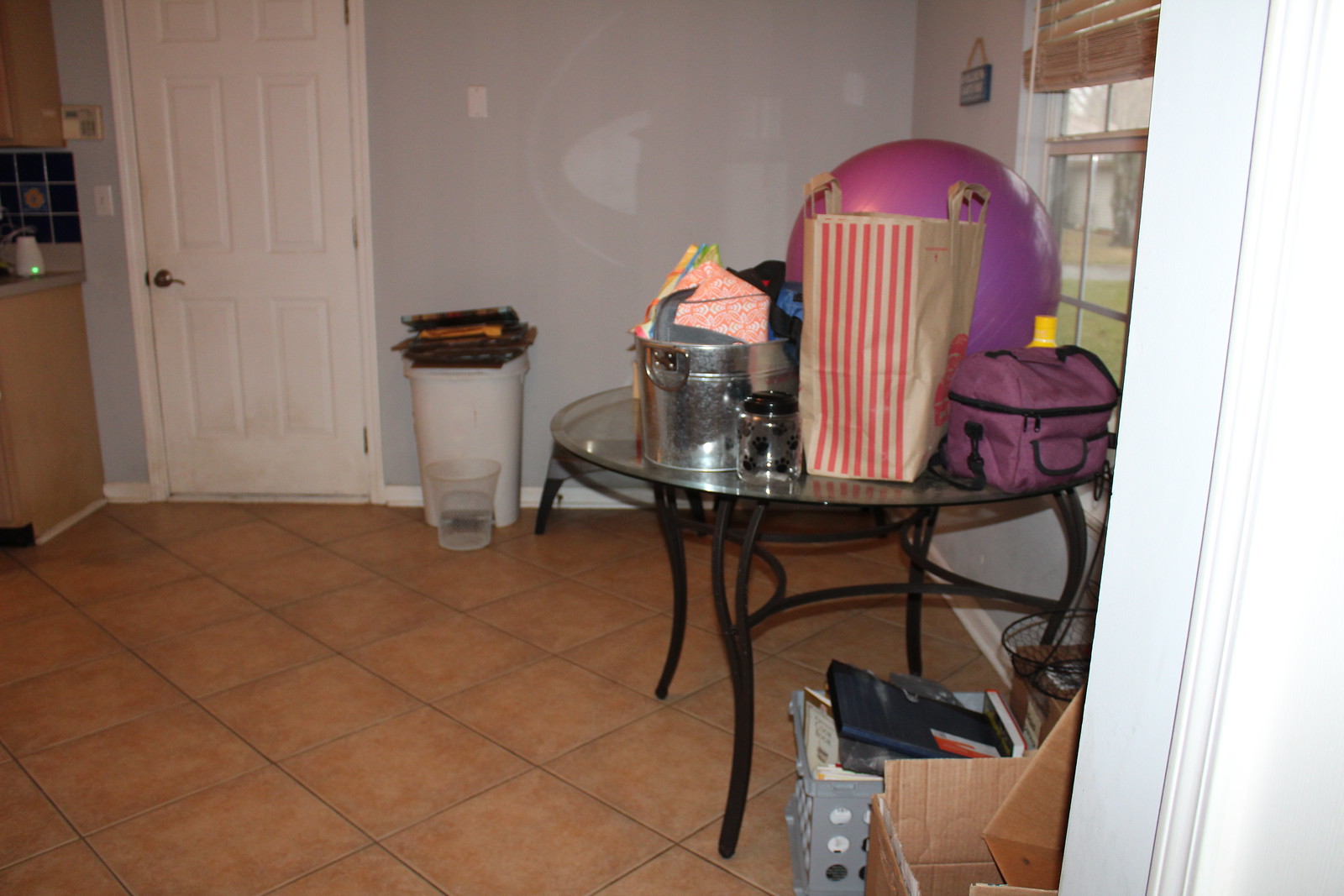A cozy kitchen characterized by a brown tile floor and gray walls. On the left side of the wall, a shut white door stands prominently. Adjacent to the door on the right, a white garbage can sits next to a bucket that is half-filled with water. Dominating the center of the scene is a glass table with elegant black iron legs. Atop the table, a purple cloth lunch bag is placed next to a distinctive see-through cup adorned with black paw prints, likely from a pet, and a silver pan with a lid. Encroaching upon the space between the paw-printed cup and the lunch bag, a white shopping bag with pink stripes is set against a backdrop cluttered with items that include a purple object, possibly resembling a hair dryer or maybe an exercise ball, obscured by other items. Adding to the organized chaos, a gray basket with holes contains various books and miscellaneous objects, while some cardboard boxes are stacked beside it.